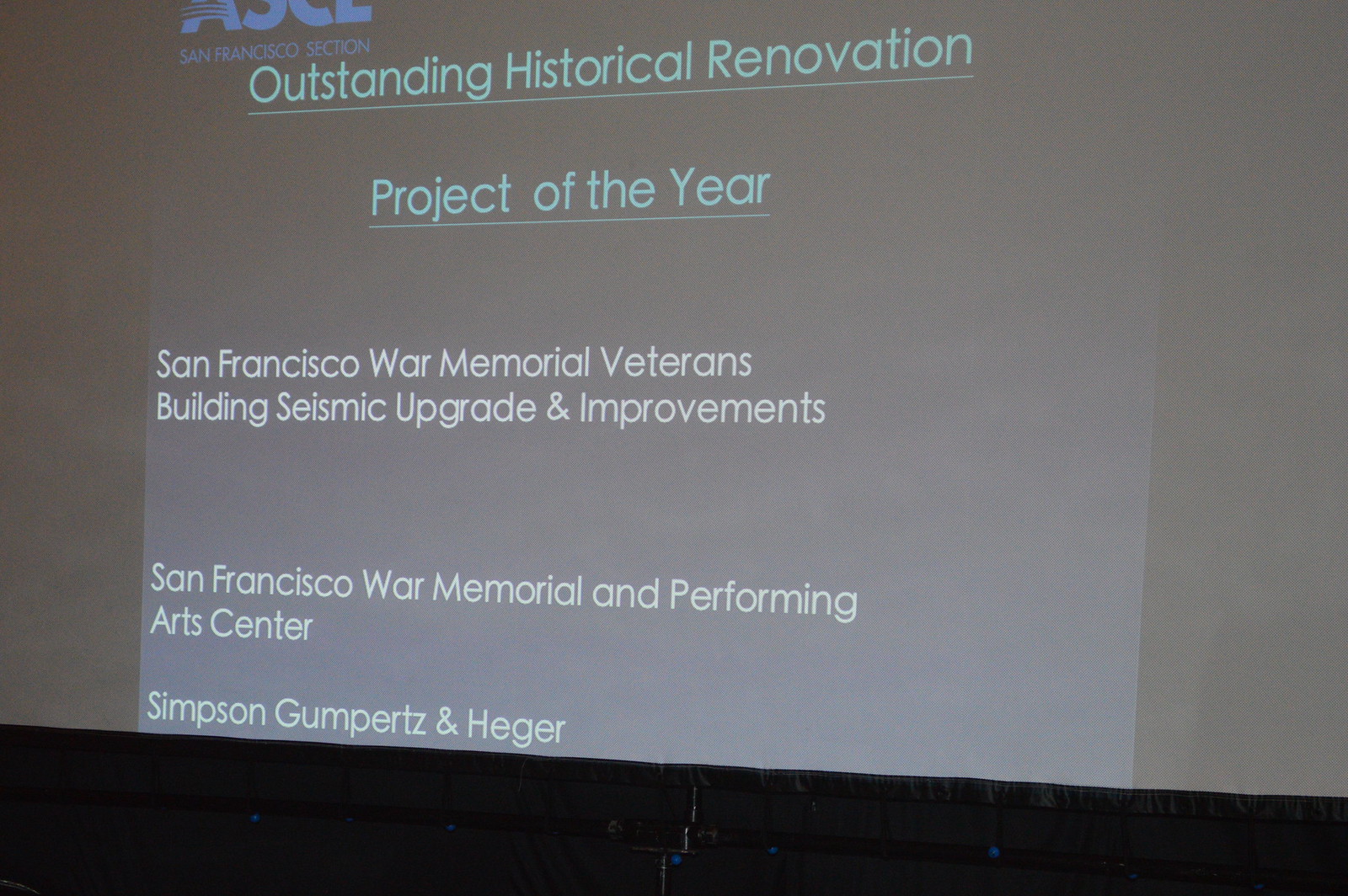The image appears to be a photograph of a large rectangular projector screen that is horizontally aligned. The bottom of the screen is dark, possibly black fabric, which suggests it might be taken on a stage. The background of the screen itself is dark gray with a medium gray center, where the text is displayed. There is a white border at the top of the screen, partially cut off and unreadable, except for a barely visible logo that may say "A-S-C-E."

Prominently under the logo, in blue text, the screen reads "San Francisco Section." Below this, the headline in blue text with an aqua underline states, "Outstanding Historical Renovation Project of the Year." Following this, left-aligned in light blue underlined text, it reads "Project of the Year." Further down in white text, it states, "San Francisco War Memorial Veterans Building Seismic Upgrade and Improvements." Additional lines below in white text read, "San Francisco War Memorial and Performing Arts Center," with appropriate spacing between the lines. Finally, at the bottom, the text "Simpson, Gumperts, and Heger" is displayed. There's no presence of people in the image, emphasizing its presentation format.